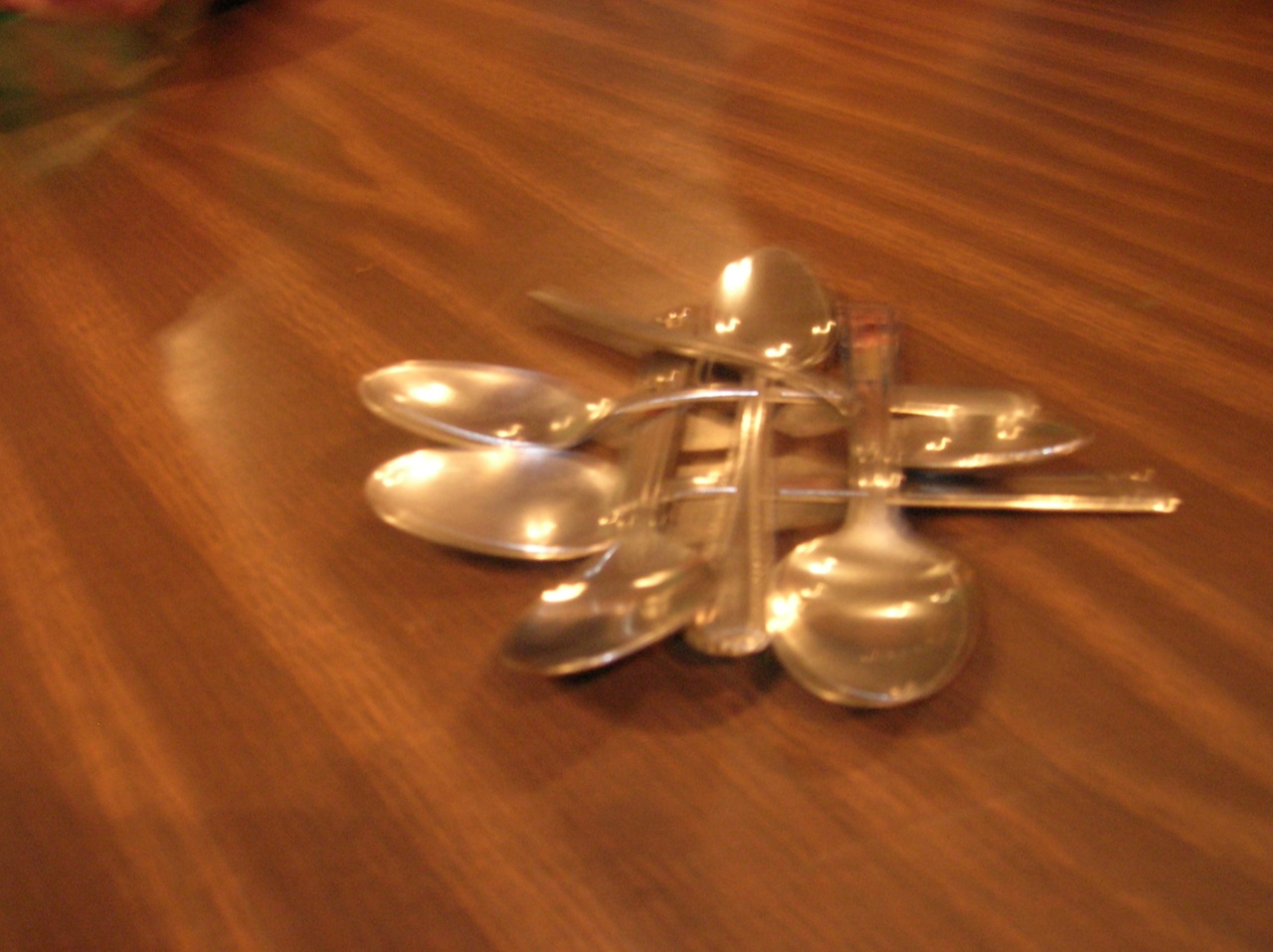This slightly blurry photo features an intricate arrangement of metal spoons stacked in a woven, lattice-like pattern on a wooden table. Approximately six or seven silver spoons, both shiny and reflective, create a layered structure that resembles a woven piece of cloth, following an over-under pattern. The spoons are aligned differently, with some facing right and others facing left, contributing to the overall circular, tangled design. The wooden surface beneath them has a noticeable grain and a laminated finish. The reflections from overhead lighting add highlights to the spoons, emphasizing their metal texture.